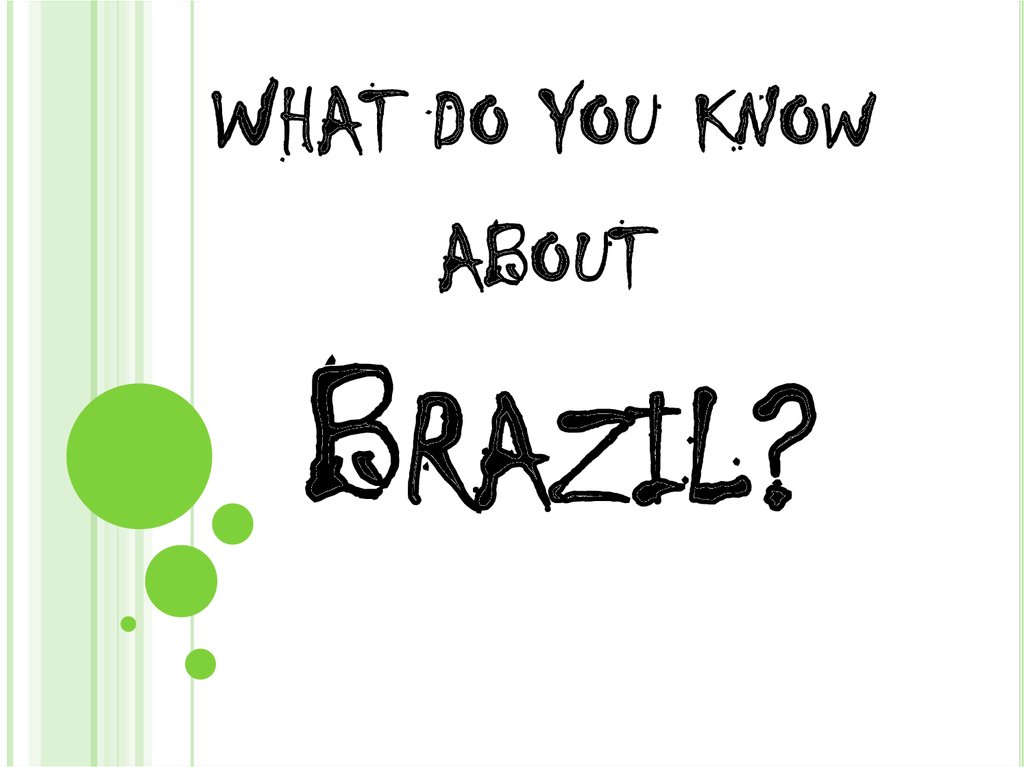This image appears to be a screenshot from a web page or possibly a banner. It features the text "What do you know about Brazil?" prominently displayed in an eye-catching, handwritten-style font. The font is digitally created to mimic organic handwriting, complete with intentional imperfections, such as occasional misplaced dots. Notably, in the word "Brazil," there's a distinctive swoosh that curls up at the bottom of the 'B,' a quirk also seen in the word "about."

The text is in black, contrasting starkly with the background to draw attention. Flanking the text on both sides are decorative elements: on the left, a series of circles in varying sizes—one large, one medium, two small, and one tiny—are arranged vertically. On the right, a simple green line descends from the top to the bottom of the image, adding to the symmetry and visual interest.

The overall design combines modern digital techniques with a touch of artisanal charm, making it both engaging and visually compelling.